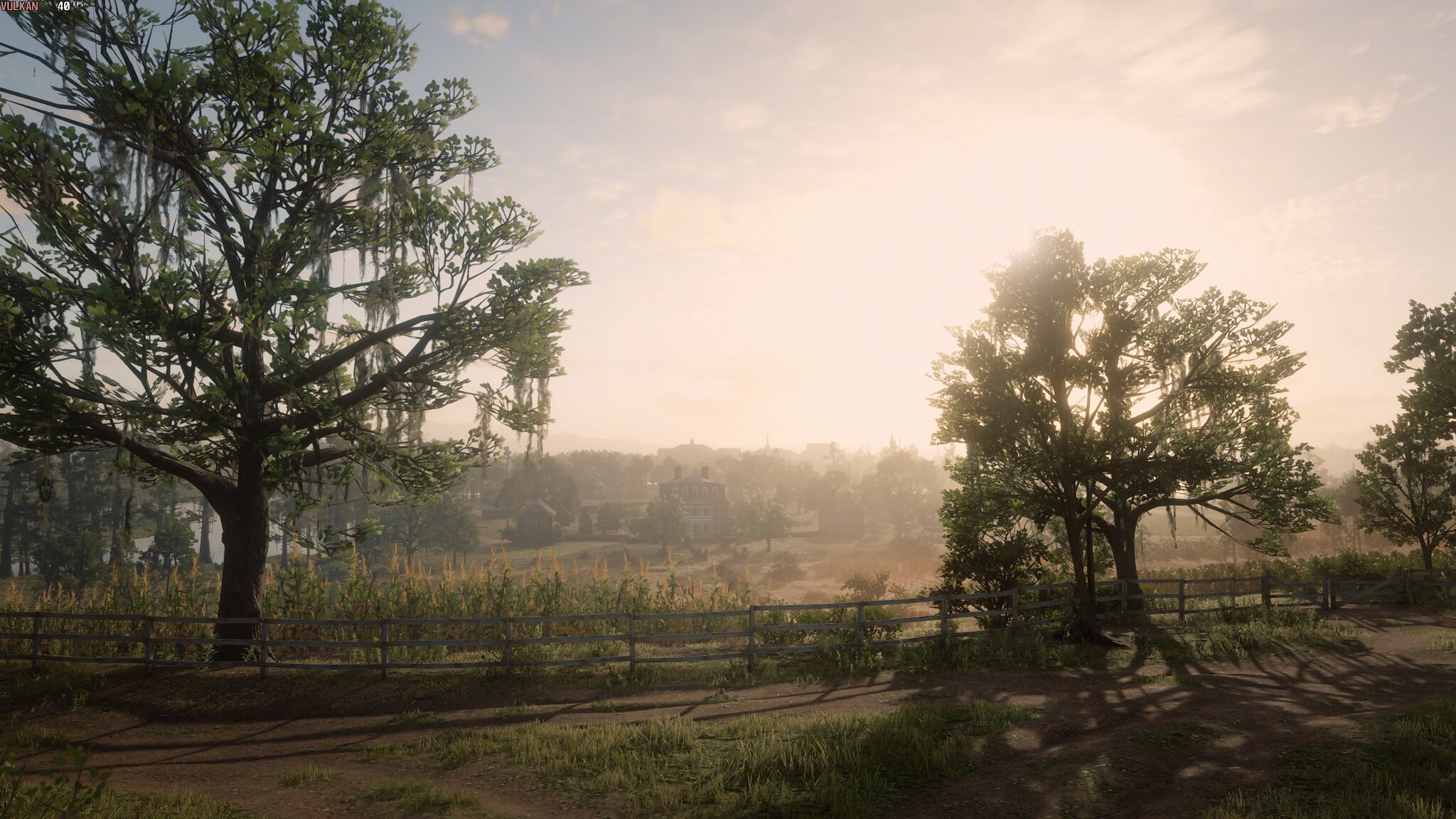This stunning outdoor scene, which could be a photograph, an AI-generated image, or even a detailed drawing, features a diverse landscape with a mix of natural elements and human habitation. Dominating the left side of the image is a large tree with verdant leaves, under a sky tinged with the light of either dawn or dusk, casting a soft, misty atmosphere over the scene. To the right of this tree, a wooden fence stretches horizontally across the entire picture. In front of the fence lies what appears to be a dirt road or pathway, and patches of green grass lay scattered throughout.

Beyond the fence, there's a sequence of trees with lush green foliage. Among these trees, further in the background, is a field potentially planted with corn or another crop. The distant horizon reveals a farmhouse or house outlined amidst the trees and greenery. The scene is wrapped in a mix of fog and sunlight, with wispy clouds adorning the bluish sky. Shadows cast by the trees fall gently on the right side of the image, enhancing the depth and calmness of this beautiful rural landscape.